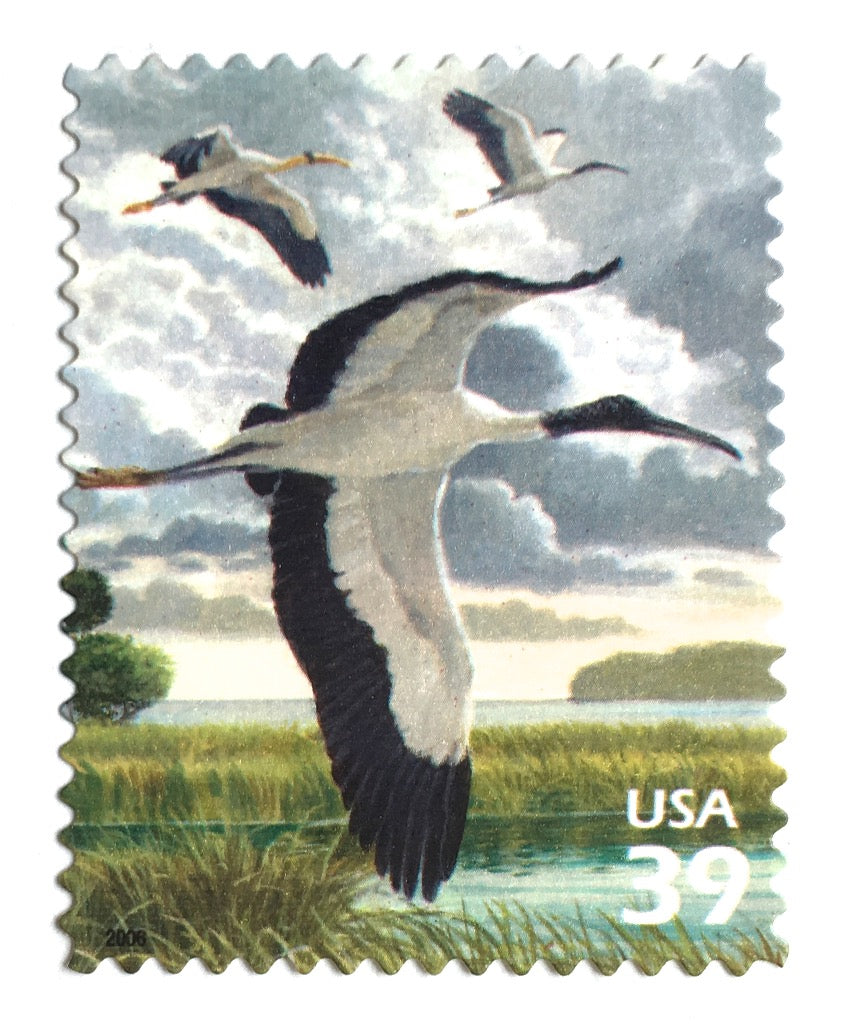In this vertically rectangular, multi-color artistic print border by zigzag patterns, we are presented with a detailed depiction of a United States of America postage stamp, valued at 39 cents. Captured on a cloudy day using natural light, the vibrant image showcases the serene beauty of nature. The focal point of the stamp features three elegant cranes, characterized by their striking black and white plumage. The center crane, noticeably larger, boasts long, extended wings with white feathers on the upper half and dark navy blue on the lower half, complemented by an orange or yellow head with a distinct black stripe. The other two cranes share similar markings, with one having a full black head.

These majestic birds soar over a calm marshland, which occupies the lower portion of the scene with its thick green grasses emerging from the water. An open lake stretches towards the middle of the image, surrounded by lush, marshy areas. In the backdrop, a layer of clouds accentuates the natural beauty of the scene, while trees in the distance hint at the expansiveness of the landscape. The lower right-hand corner of the stamp is marked with "USA" and the denomination "39," indicating its value as a piece of historical postage.